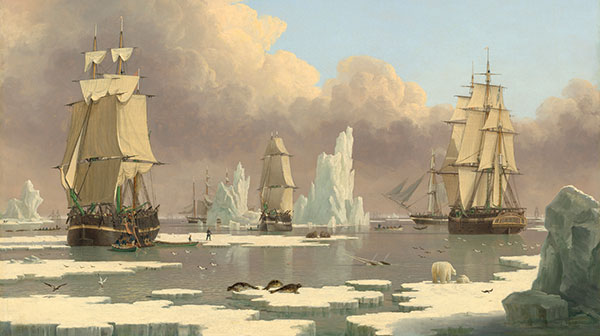The image is a detailed, black and white drawing of a historic scene, most likely from the late 1800s, depicting five to seven sailboats navigating icy waters, which may be in Antarctica. The water is cluttered with icebergs and floating ice pieces, with some hosting polar bears and seals. The scene includes active seabirds and penguins dispersed throughout the ocean and on the ice. Additionally, there are two people walking on the ice in the distance. The sky, painted in blue with dense grey and dark grey clouds, forms a contrasting backdrop to the black and white setting. The overall lack of color, except for the blue sky, enhances the stark and frigid atmosphere of the environment.